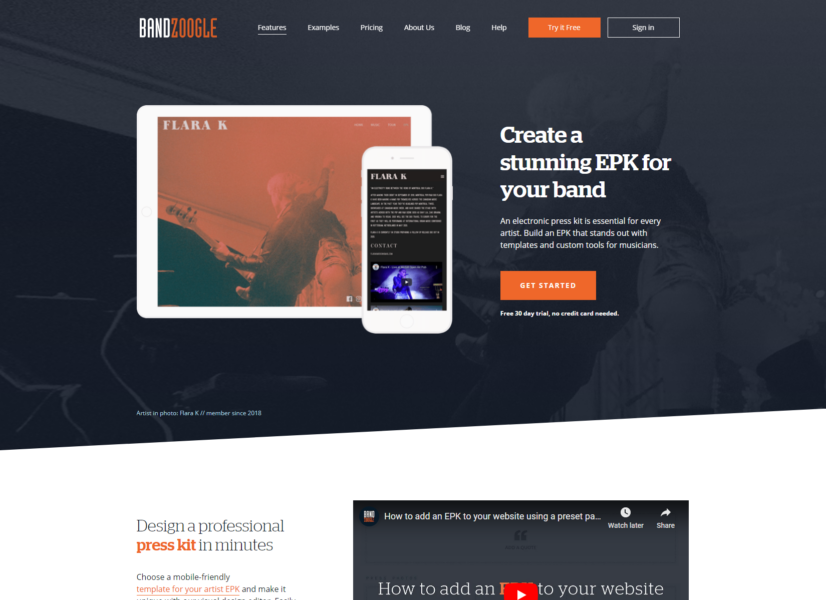The image features a white background, prominently showcasing the website navigation options, which include:

1. Bandzoogle
2. Videos (Vidges)
3. Examples
4. Pricing
5. About Us
6. Blog
7. Help
8. Try It for Free

Directly beneath these options, there is a "Sign In" button.

An iPad display below these navigational elements features an interface with the following details:

- The username "Flora Kay" is shown in red.
- Promotional content such as "Purchasing the Shows" and "Create a Stunning APK for your Band."
- A message that an Electronic Press Kit (EPK) is essential for every artist.
- Instructions to build an APK that stands out, using templates and custom tools for different positions.

A prominent rectangle on the display contains the text:

- "Get Started"
- "Free 30 Day Trial"
- "No Credit Card Needed"

Adjacent to this is a smartphone screen again showing "Flora Kay," suggesting it is a user interface or user-centric feature. There is accompanying text implying a human presence, with the text "Video."

Further down is additional instructional content:

- "Design a Professional Press Kit in Minutes"
- "Choose a Mobile-Friendly Template for Your Artist APK and Make It"

A video tutorial interface is displayed with a description: "How to Add an APK to Your Website Using Preset." Options available include "Watch," "Letters," and "Share."

The central part of this video interface shows a red square alongside a wide, sideways triangle, indicating play or media controls typically associated with a video player.

Overall, the image seems to depict an online platform focused on helping artists create and manage electronic press kits (EPKs) with various tools and templates, alongside promotional offers for a free trial.